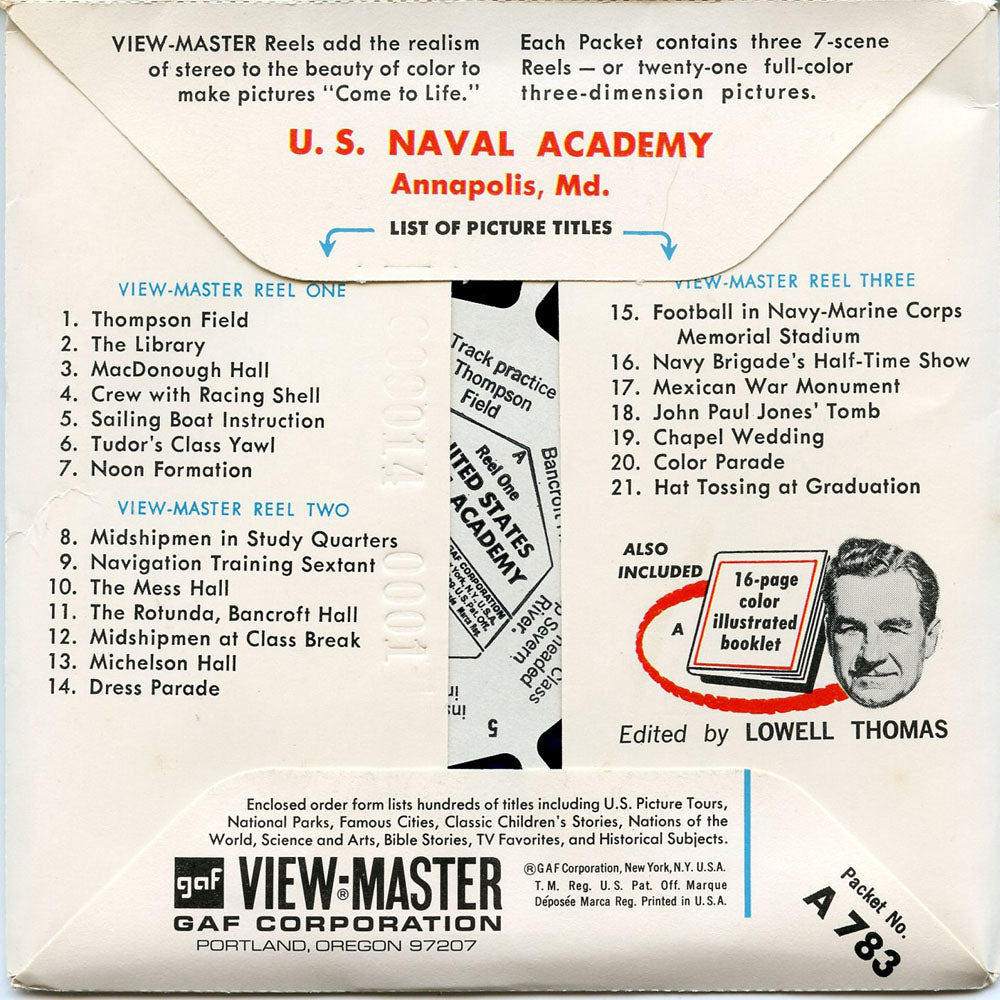This image depicts the backside of a vintage Viewmaster reel packet from the 1970s, specifically themed around the U.S. Naval Academy in Annapolis, Maryland. The packet is square, resembling the back of a CD or disc holder, and features numerous black text details across its surface. At the top, where the flap folds over, bold black text reads, "Viewmaster," followed by the promotional slogan, "Reels add the realism of stereo to the beauty of color to make pictures come to life." Under this, the packet highlights that it contains three seven-scene reels, totaling 21 full-color, three-dimensional pictures. Prominently in large red letters, it says, "U.S. Naval Academy, Annapolis, MD," below which a section titled "List of Picture Titles" is displayed. This list is organized into three columns for each reel: "Viewmaster Reel 1," "Viewmaster Reel 2," and "Viewmaster Reel 3," with detailed scene titles listed for each reel, from 1 to 21. On the right-hand side, there's an image of a man identified as Lowell Thomas, next to a note that states the inclusion of a "16-page color illustrated booklet, edited by Lowell Thomas." Towards the bottom of the packet, more black text includes details about the manufacturer, "Viewmaster GAF Corporation," and the packet number "A783." The overall appearance of the packet, its listed contents, and detailed descriptions hark back to a nostalgic era of the Viewmaster toy, a popular small film rotator that used round picture discs to display stereoscopic images.